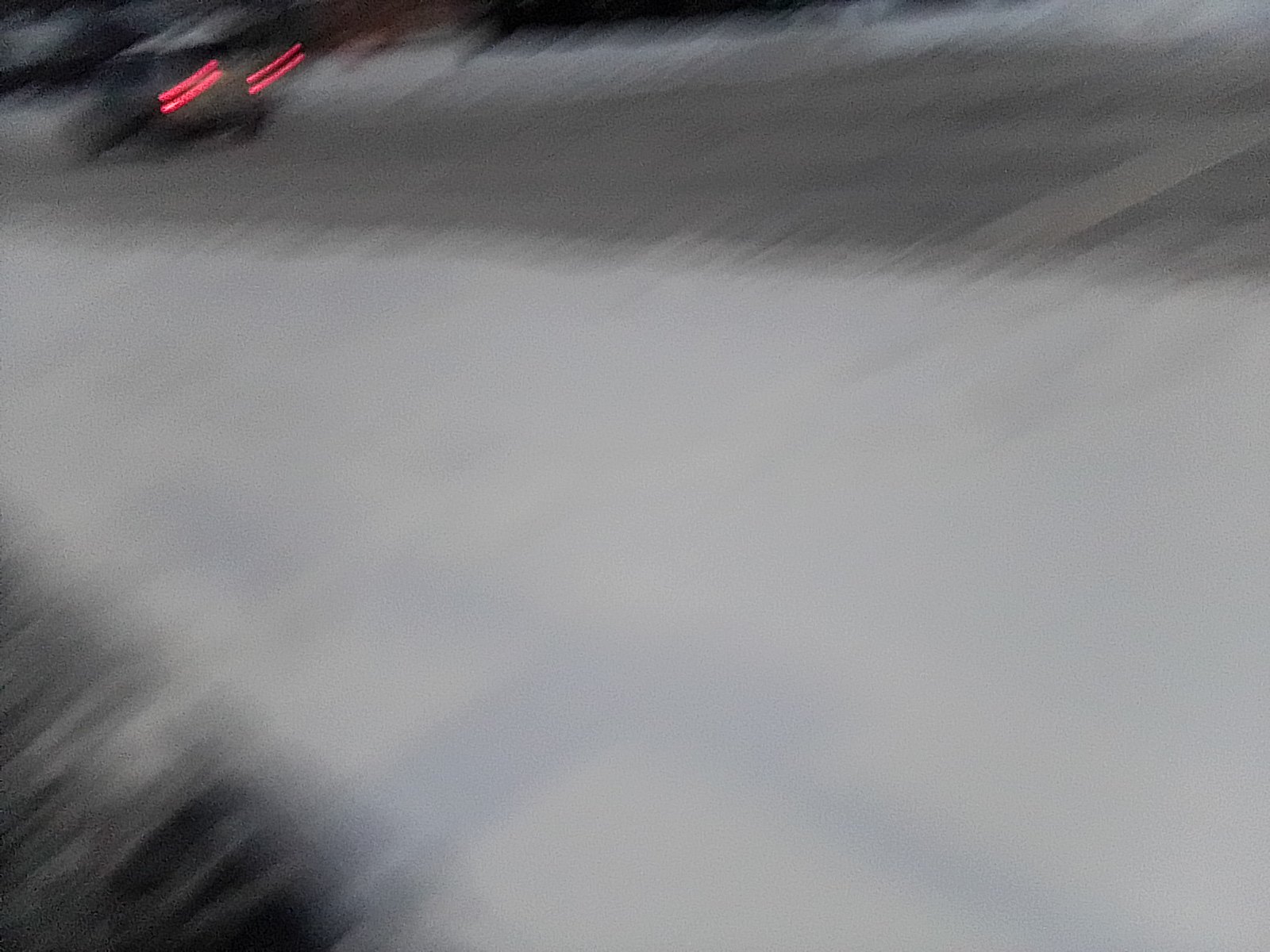A blurred, panoramic image captures a winter scene of traffic in motion. The composition suggests the photo was taken outdoors on a cold, winter day, possibly while moving. Dominating the lower portion is a thick swath of white, likely indicating snow, diagonally stretching from the bottom right to the left side of the frame. Contrasting this, the bottom left corner is dark. The upper segment of the image features a road running horizontally, where the back of a car is visible on the left side. The car's red taillights form two parallel pairs of glowing lines, accentuating the motion blur effect. Despite the wintry conditions, the road itself appears mostly clear of snow. Overall, the image exudes a sense of dynamic movement amidst a frosty, blurred backdrop.